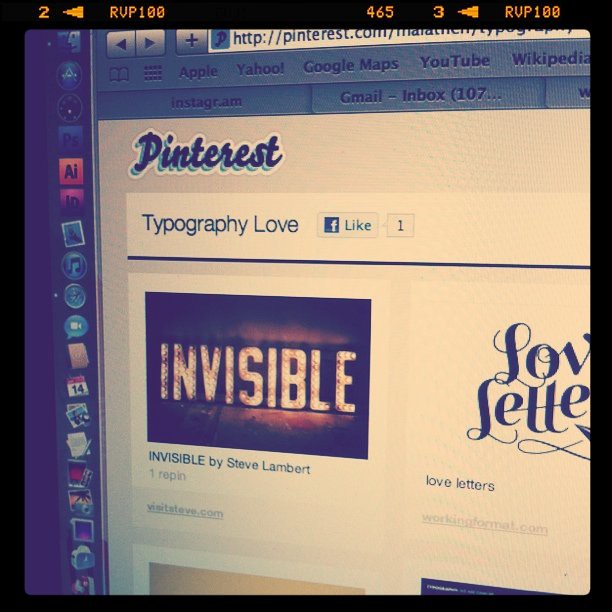The image is a photograph of a computer screen, bordered in black. At the top of the screen, yellow text reads "2" followed by a yellow triangle pointing left, "RVP 100," while more to the right it states "465 3" with another left-pointing yellow triangle and "RVP 100." The central focus of the screen is a Pinterest page titled "Typography Love" in blue letters, featuring numerous images related to the topic. Prominently displayed is a darkened rectangle with "Invisible" written in bold font, attributed to Steve Lambert. On the left vertical edge of the screen are about 10 to 15 icons, including recognizable ones like a video camera, the date, and an AI symbol in black font on a red background. The overall scene is cluttered with various visual elements indicative of active browsing and usage.